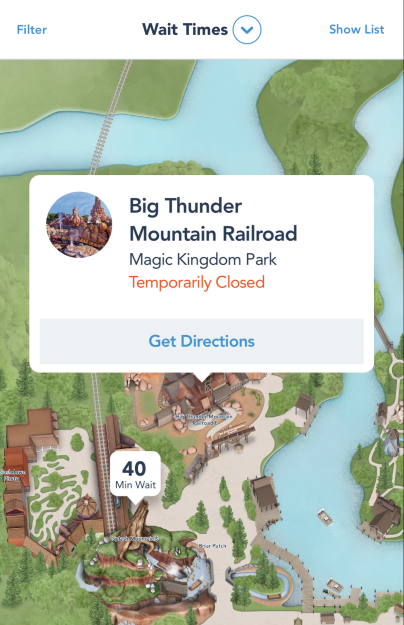This vertically oriented image appears to be a screenshot from the Disney World app, displaying wait times for various attractions across the different Disney theme parks. Dominating the background is an aerial view of the Magic Kingdom, showcasing its distinctively blue waters and lush green areas where the rides are situated. On the right-hand side of the image, a thin black vertical line runs from top to bottom, while the other edges remain borderless.

At the top-left corner, the word "Filter" is displayed in blue text, accompanied by the central heading "Wait Times" in black text, which features a blue circle with a downward-facing arrow. Positioned at the top-right, "Show List" is also highlighted in blue.

Centrally, the user has selected a specific attraction, revealing a pop-up box. This box shows a wait time of 40 minutes and features a smaller inset that displays information about Big Thunder Mountain Railroad. The attraction is indicated as "Big Thunder Mountain Railroad" in black text, followed by "Magic Kingdom Park" in orange text indicating it is "temporarily closed." Below this, a gray box provides an option in blue text to "Get Directions." 

Overall, the image successfully conveys key information about ride wait times and the operational status of specific attractions, set against the visually engaging backdrop of the Magic Kingdom.